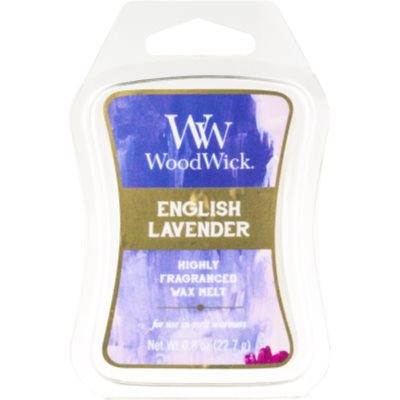The image features a pristine, brand-new package of WW Woodwick English Lavender Highly Fragranced Wax Melt, centrally positioned against a stark white background. The object is housed in a curvy rectangular, clear plastic blister pack, which includes a hang tab hole at the top for display purposes. The design elements on the label feature an abstract blend of colors: dark blue at the top transitioning into lighter blue and purple, with accents of pink and gold. The text on the label is clearly legible, with "WW" and "Woodwick" in staggered white text at the top, followed by a gold label in the center stating "English Lavender." Below that, the label indicates "Highly Fragranced Wax Melt" in white text. There is a hint of red in the bottom right corner of the label, adding to the detailed, visually appealing packaging. The item's careful presentation and the clean, professional style of the image make it look like a typical product photo one might find in retail settings such as Bed, Bath and Beyond.